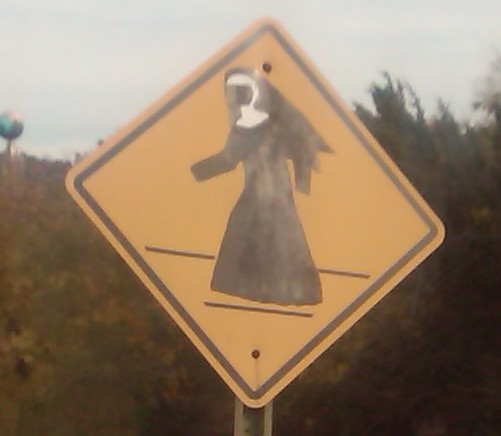In the photo, a gray sky looms over the upper third of the image, casting a somber tone over the scene. Below the sky, a blurred brown hill stretches across the middle of the photo, dotted with sporadic trees to the right and scattered bushes throughout, creating a rural Midwestern landscape. Centered prominently in the photo stands a metal rod emerging from the ground, supporting a yellow diamond-shaped road sign. The sign, outlined with a bold black border, displays an unusual figure—a nun dressed in a long black habit and white headdress—walking leftward. The sign is evocative of a typical pedestrian crossing sign but intriguingly altered with the distinctive nun figure, adding a peculiar twist to the otherwise serene setting.